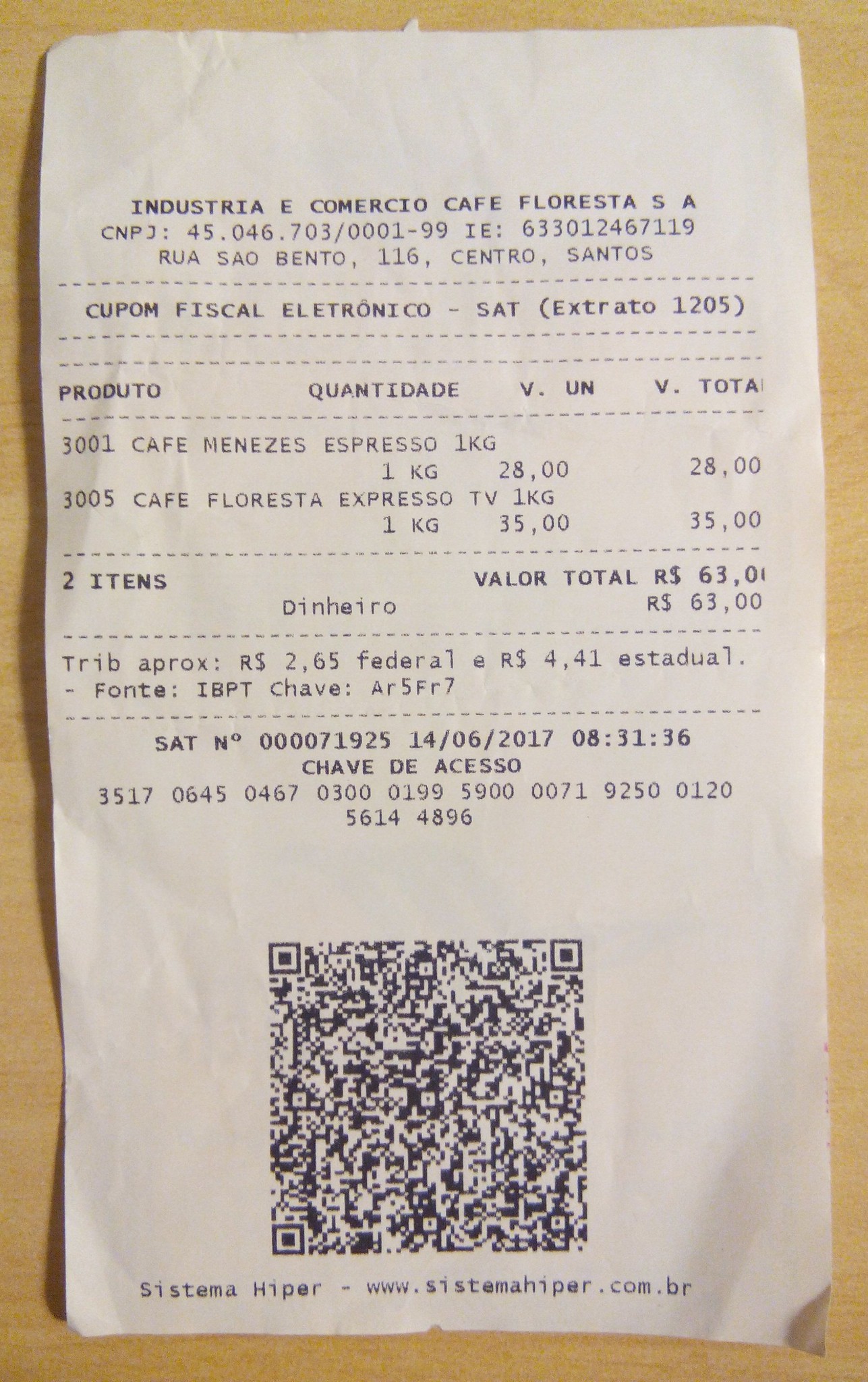Receipt from *Industria y Comercio Cafe Floresta S.A.* on a white or beige wooden surface:

1. **Header Details:**
   - *Industria y Comercio Cafe Floresta S.A.*
   - Contact Information beneath the café’s name.
   - Notation in Spanish: *CUPAM Fiscal Electronico*.

2. **Itemized List of Purchases:**
   - Separated by dotted lines.
   - Columns detailing product numbers, item names, and numerical totals.

3. **Transaction Summary:**
   - States the total count of items: *2 items*.
   - An additional section potentially referencing taxable amounts.

4. **Footer Information:**
   - Date: *14-06-2017*.
   - Time: *08-31-36*.
   - Group series of four numbers.

5. **Barcode and System Information:**
   - A scan code.
   - Website: *Sistema Hyper* - www.sistemahyper.com.br.

The receipt, small and white, lies flat on a clean, light-colored wooden surface, accentuating the simplicity and clarity of its details.